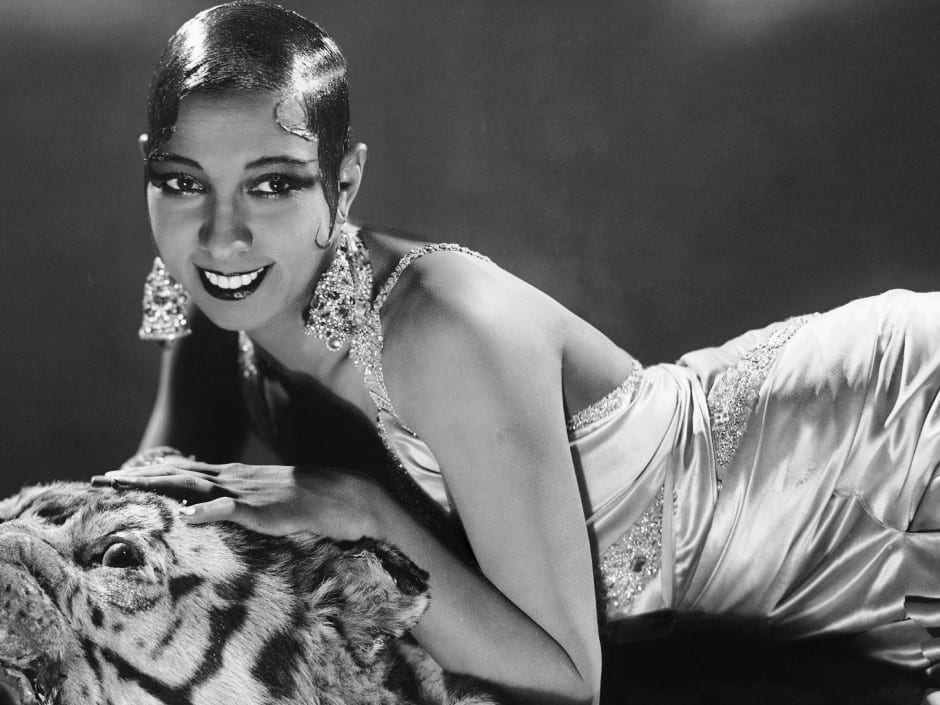This black-and-white photograph captures a woman, potentially an African American, modeled in the style of the 1920s flapper era. She lies on her stomach with her arm resting on what appears to be the head of a tiger, likely part of a tiger throw rug, as the rest of its body is not visible. Her attire is a sleek, sleeveless dress that has a satin or silk sheen, adorned with jeweled or diamond-like patterns around her chest and belly area. She has large, triangular metallic earrings that dangle prominently, resembling Christmas trees covered in jewels. Her makeup is bold, featuring darkly shaded eyes and dark lipstick. Her hair is slicked down with product, styled into shiny, immovable curls and wave patterns at the front and sides. The background is a plain, darkish-gray, lending an old-school, vintage feel to the image, reminiscent of early 20th-century portraiture.